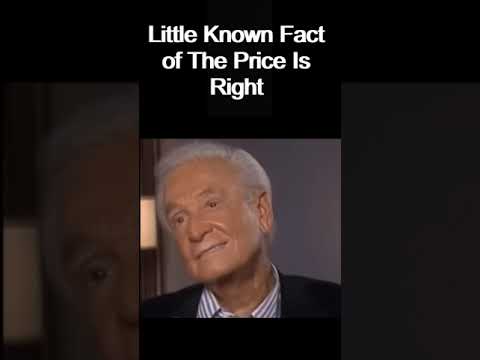The image features an elderly Bob Barker with completely white hair, looking off to his right with his head slightly tilted and a faint smile showing a hint of teeth. He is dressed in a blue and white striped collared shirt beneath a black jacket. Above him, the text "little known fact of the price is right" is prominently displayed in white letters against a black background. The image itself is presented in portrait mode with a square aspect ratio, and the background is a dark, gray-tinted enlarged version of the top portion of Bob Barker's face, placed on the left side of the screen. The right third of the screen is filled with a plain gray wall, enhancing the focus on Barker's visage. The overall composition juxtaposes the smaller, centered portrait with the larger background, adding a layered depth to the photograph.